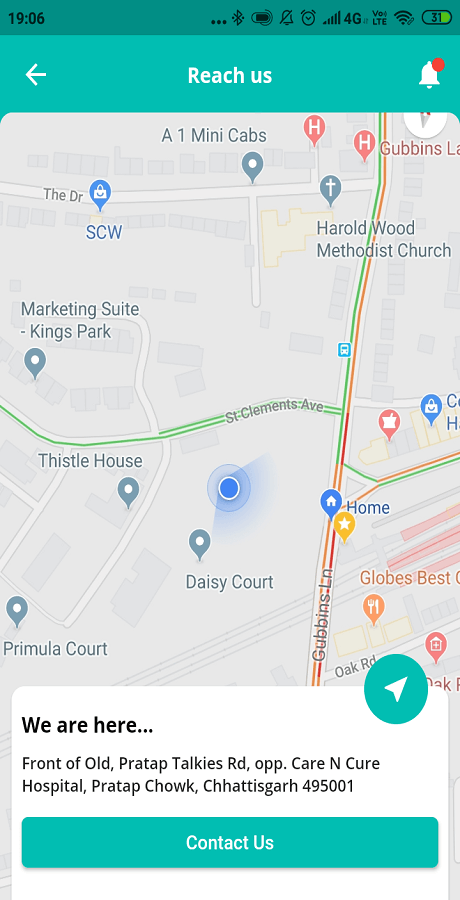A detailed and clean caption for the image would be:

"The image shows a cell phone screen displaying a map. At the top of the screen, a dark teal bar contains various status icons and information, including the time '19:00' on the left, and icons for cellular signal strength, Bluetooth, sound off, alarm, 4G connectivity, Wi-Fi signal, and a battery level at 31%. Below the dark teal bar, there's a lighter teal bar featuring a back arrow on the left, the text 'Reach Us,' and a bell icon with a red notification circle, all in white. 

The main portion of the screen displays a map indicating a location. Beneath the map, there is a text box with the heading 'We Are Here' and the address details: 'Front of Old Pratap Talkies Road, Opp. Care and Cure Hospital, Pratap Chowk, Chhattisgarh, 495001.' At the bottom of the screen, there is a large, dark turquoise button labeled 'Contact Us.' Additionally, on the right corner above the white pop-up that obscures part of the map, there is a white circle with a triangle inside it. The Care and Cure Hospital is not visible in the image."